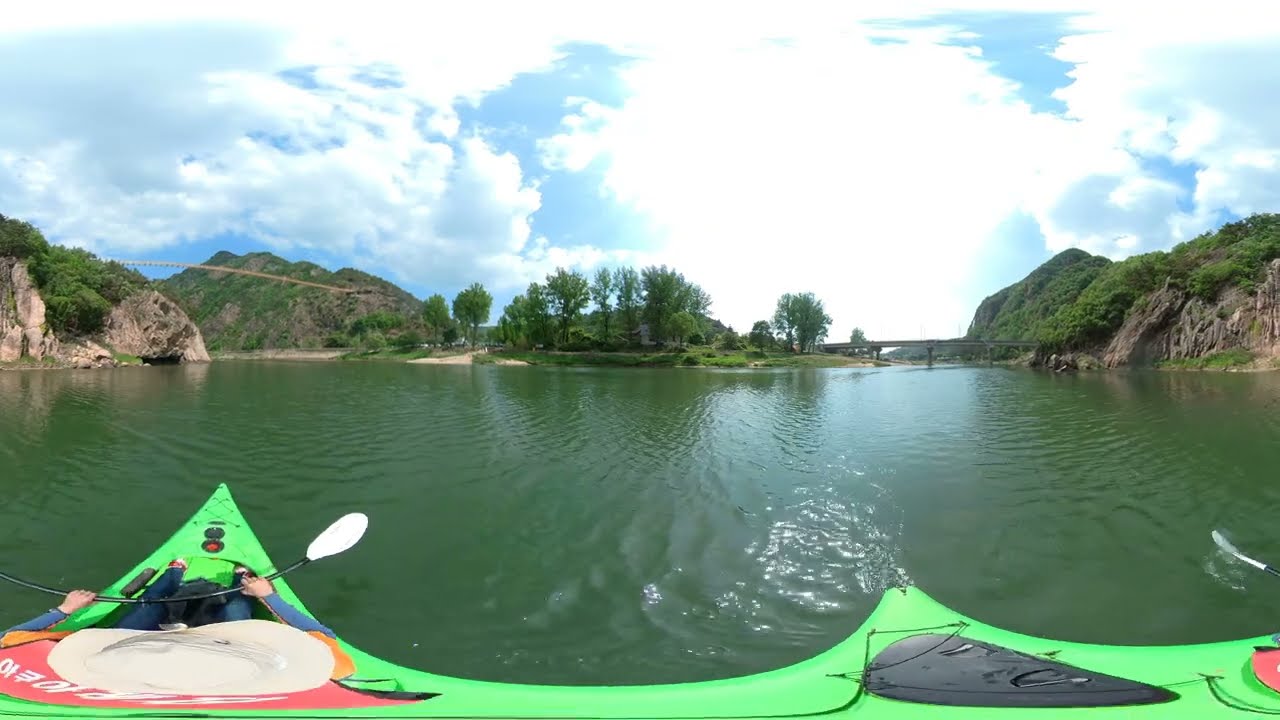This panoramic 360-degree image captures a serene scene of a person kayaking on a calm, dark green body of water, possibly a lake or river. The person is in a bright lime green kayak, wearing a blue outfit and a hat, and can be seen holding a black oar with white paddles across their body. The kayak occupies the central part of the image, with the water stretching out to the left and right, appearing clear but distinctly green.

In the background, the viewer can see low rocky cliffs adorned with sparse greenery and some areas completely bare. Centrally located beyond the kayaker is a much greener hill populated with numerous trees. Additionally, to the right in the far distance, there is a faint view of a bridge crossing the water.

The sky above is vast and blue, filled with an abundance of white and light gray puffy clouds, adding to the tranquility and expansive feel of the scene. The combination of green water, rugged cliffs, greenery, and a vibrant sky creates a picturesque and immersive visual experience.